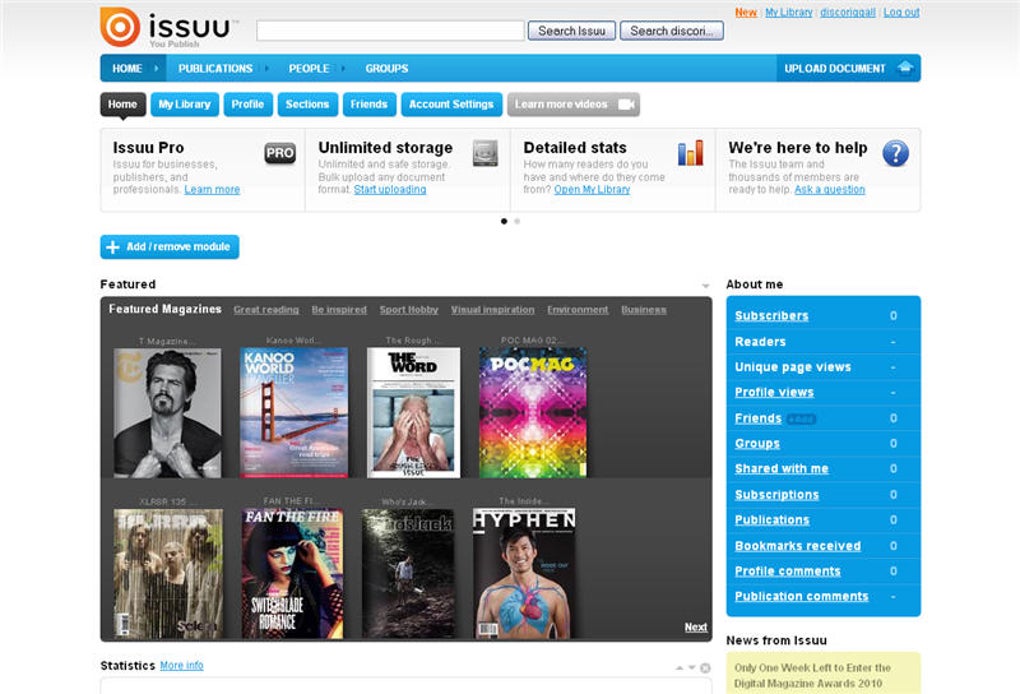The webpage features the 'Issuu' platform, prominently branded at the top with its name, "ISSUU," and an accompanying orange logo to the left. Adjacent to the logo is a search bar labeled to facilitate searches within "Issuu" and "Discovery," both encapsulated in gray boxes. To the right of the search bar, the interface displays the word "New" in orange, followed by "My Library" in blue.

Beneath the primary navigation, there is a blue navigation bar offering multiple options: "Home," "Publications," "People," and "Groups," allowing users to explore different sections of the platform. Users also have the option to upload documents from this section.

Further down, a black box provides more personalized navigation options, listing "Home," "My Library," "Profile," "Sections," "Friends," and "Account Settings," each associated with blue buttons to click on.

To the side, there is a section for education and storage, labeled "Learn." This includes "Learn More Videos," "Unlimited Storage," and "Detailed Stats." A help section is accessible via a question mark icon. Below this, a blue "Add or Remove Module" bar is present.

Beneath these elements lies a grey box displaying thumbnails of various magazines or digital CDs. On the right side of the page, a blue box provides a detailed "About Me" section, featuring metrics and user engagement statistics such as "Subscribers," "Readers," "Unique Page Views," "Profile Views," "Friends," "Groups," "Shared with Me," "Subscriptions," "Publications," "Bookmarks Received," "Profile Comments," and "Publication Comments." Each of these categories is organized within the blue box for easy navigation and reference.